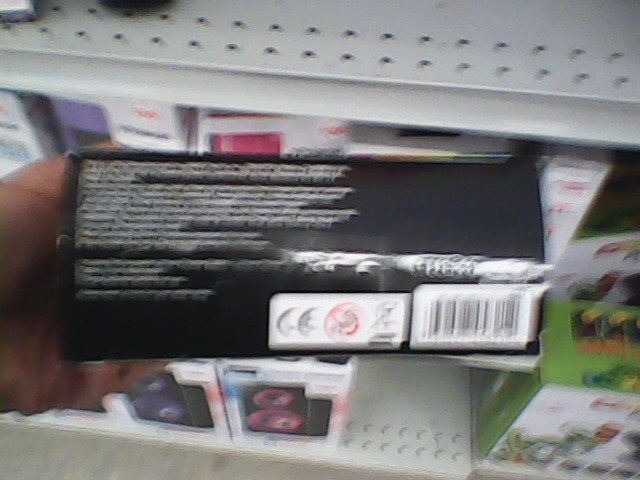In this very blurry image, a Caucasian hand is holding a black rectangular cardboard box in the foreground of a store aisle. The black box has unreadable white text on the left side and a white rectangle with a barcode and another smaller white rectangle containing symbols on the bottom right. The scene is set against white metal shelving units with small holes. On the top shelf, partially cropped out, an object is visible. The bottom shelves are stocked with various boxes; to the left, there are white boxes depicting black speakers with colorful accents, possibly stereos, while the right side features white boxes accented with green. This image captures the intimate detail of a retail environment, focusing on a product being inspected closely.